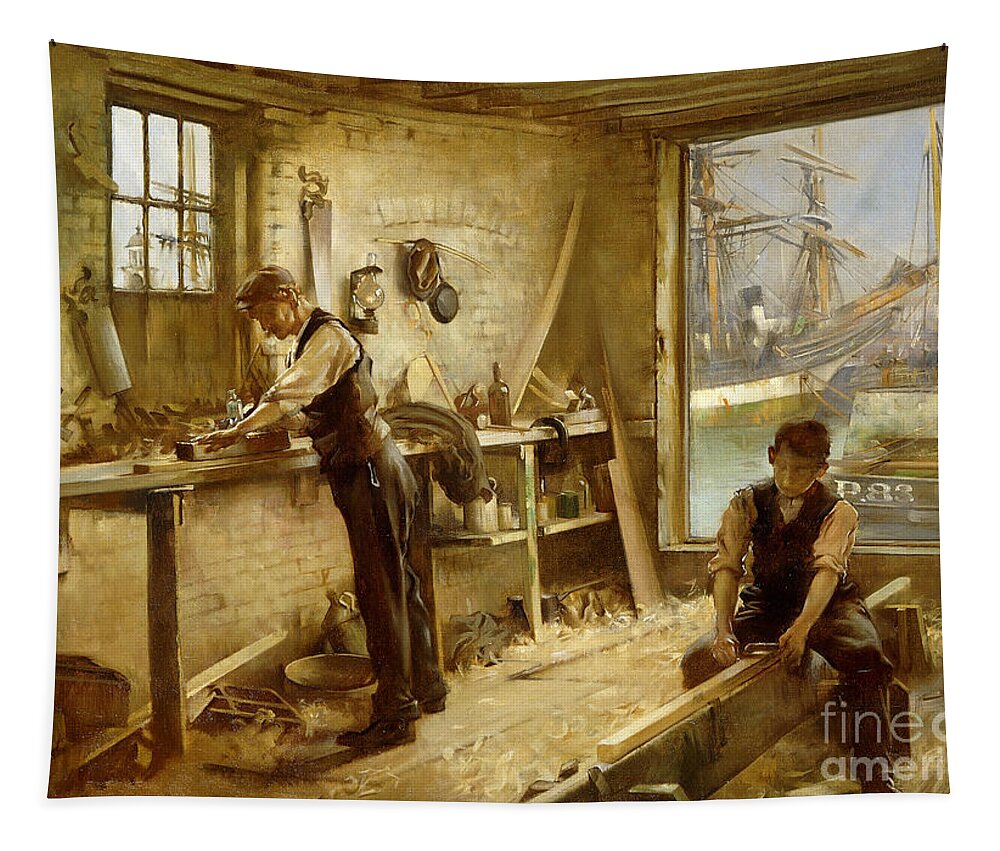The illustration depicts an old-fashioned 19th-century workshop bustling with activity. The entire scene is tinged with a yellowish hue. On the left, an older man dressed in dark brown pants, a matching vest, and a white shirt with rolled-up sleeves meticulously works on a piece of wood, surrounded by tools like saws, sawdust, and wood shavings scattered about. To the right, a young apprentice sits on a bench working on a long plank of wood, indicative of shipbuilding. The background reveals a busy harbor through a large doorway and a smaller six-paned window. Visible are tall masted ships, including a prominent blue, white, and yellow ship, alongside another ship marked "P83." This detailed artwork captures the essence of a bygone era, offering a glimpse into the intricate craftsmanship and maritime activity of the time.